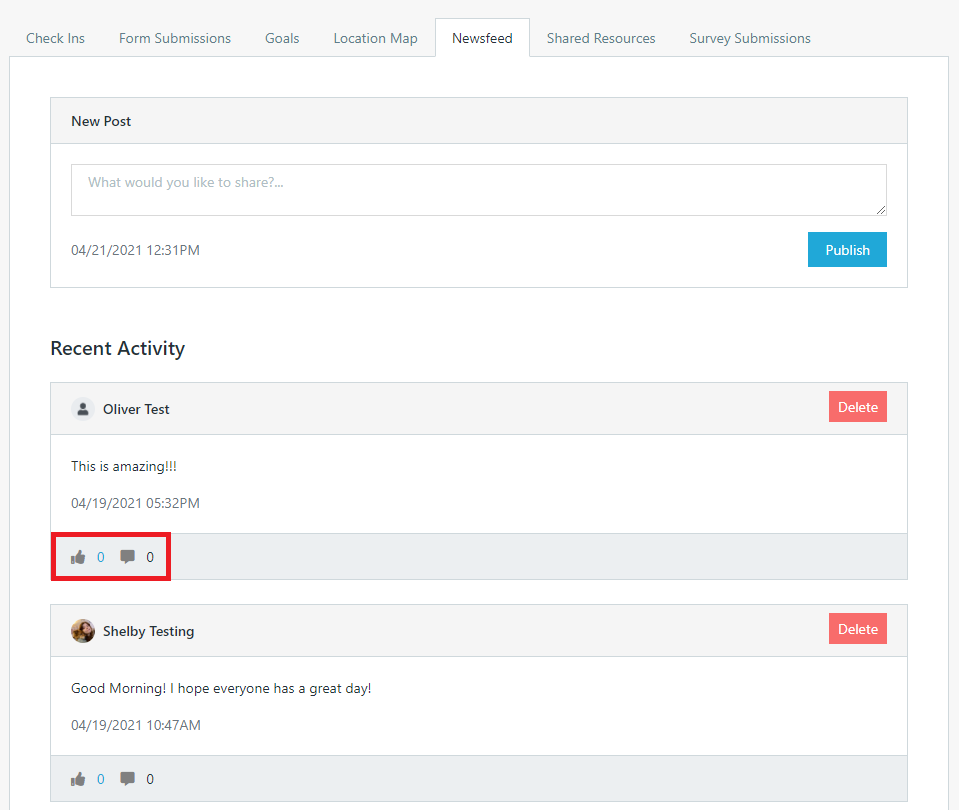The image features a predominantly white background with a substantial amount of text. At the top, there is a light gray border containing navigational options which include: "Check-ins," "Form Submissions," "Goals," "Location Map," and "Newsfeed," all in white text. The "Newsfeed" option is highlighted. 

Directly below this border is a gray rectangular section labeled "Shared Resources and Survey Submissions." Following is another gray rectangle bearing the label "New Post." Within this area, there is a text box that prompts, "What would you like to share," accompanied by the date "04/21/2021 12:31 PM."

To the right of the text box is a blue rectangle with the word "Publish" inscribed on it. Underneath, the heading "Recent Activity" is displayed.

The first entry in the activity feed shows a circular icon with a silhouette of a person's head and shoulders labeled "Oliver Test." To the far right of this entry is a red rectangle with the word "Delete." Below, it states: "This is amazing 04/19/2021 05:32 PM." Accompanying this are a red-bordered thumbs-up icon and a speech bubble, both marked with a zero.

The subsequent entry features another grey rectangle with a circular photo of a person labeled "Shelby Testing." To the far right, there is a red "Delete" rectangle. Below the entry, it reads: "Good morning. I hope everyone has a great day. 04/19/2021 10:47 AM."